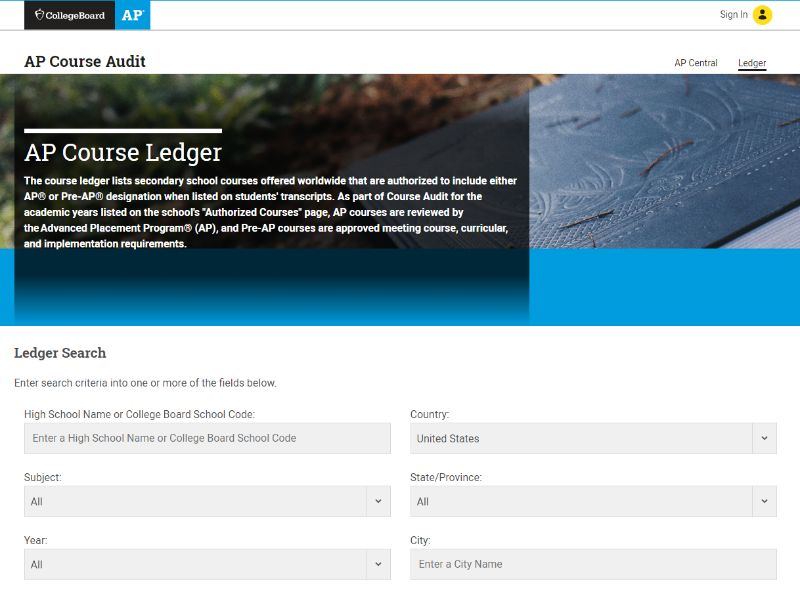The image is a screenshot of an online educational platform, specifically a section from the College Board's Advanced Placement (AP) course audit and ledger tool. At the top, the College Board logo appears on a black rectangular background next to the "AP" logo on a blue square, delineated by a thin blue line across the very top of the page. In the upper right corner, there is a "Sign In" option next to a yellow circle with a black person icon inside.

Below the top section, the page title "AP Course Audit" is prominently displayed in bold on the left, while on the right, there are links labeled "AP Central" and "Ledger," with "Ledger" being underlined to indicate it is the selected section.

Central to the page is a large photograph with a white bar overlayed, containing the text "AP Course Ledger" in white. The description below this heading explains that the AP Course Ledger lists secondary school courses offered worldwide that are authorized to include either AP or Pre-AP designations when listed on students’ transcripts.

Beneath the photo, a bright blue bar spans the width of the page, followed by a thicker, equally bright blue bar underneath.

The bottom half of the webpage is white and is titled "Ledger Search." It contains search fields organized into two columns. The left column includes:
1. "High School Name or College Board Code" with a placeholder prompting to "Enter a high school name or College Board school code."
2. "Subject," prefilled with "All" and featuring a drop-down arrow for selection.
3. "Year," also prefilled with "All" and a drop-down arrow for further selection.

The right column includes:
1. "Country," prefilled with "United States" and a drop-down arrow for other selections.
2. "State/Province," prefilled with "All" and a drop-down arrow for selection.
3. "City," with a placeholder prompting to "Enter a city name."

These search fields allow users to locate AP courses offered by various secondary schools, filtering the information based on different criteria like school name, subject, year, country, state/province, and city.